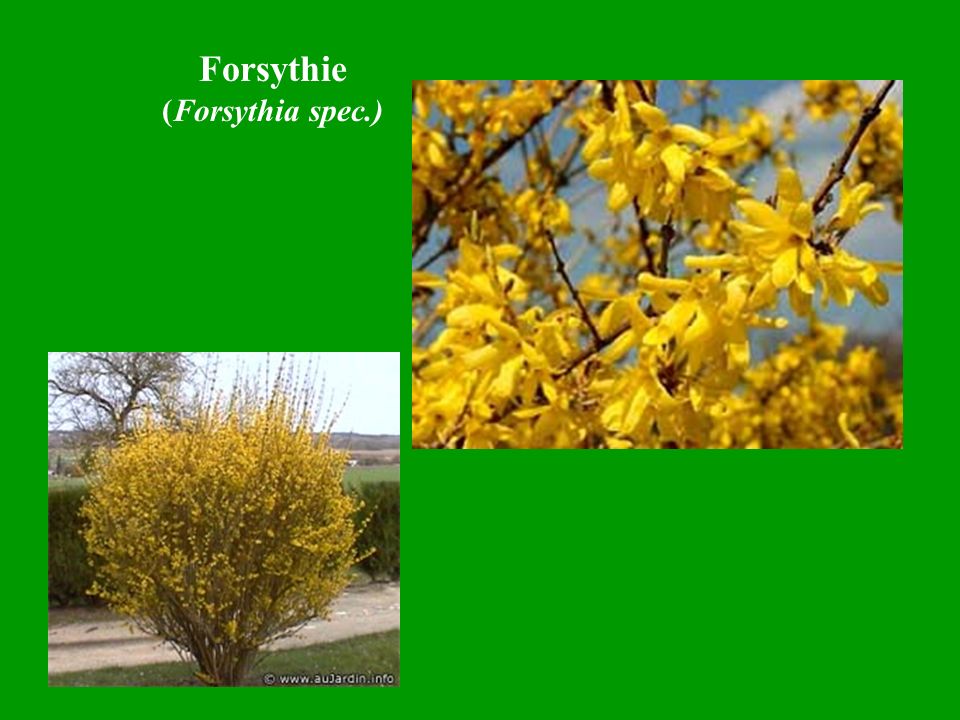The image features a green rectangular background with two embedded pictures: one in the lower left and one in the upper right. In the upper left corner, white text reads "Forsythia (F-O-R-S-Y-T-H-I-A)". Below it, in parentheses, is "Forsythia spec. (F-O-R-S-Y-T-H-I-A space S-P-E-C period)". The lower left picture provides a pulled-back view of a yellow-flowered Forsythia bush, situated next to what seems to be a dirt road or driveway with hedgerows and a horizon line in the background. The upper right picture offers a closer perspective, highlighting the individual yellow flowers of the bush with reddish-brown centers, set against a blue sky with clouds. Additionally, one of the images has the text "www.aujardin.info" at the bottom, possibly indicating an educational or commercial website related to the plant.